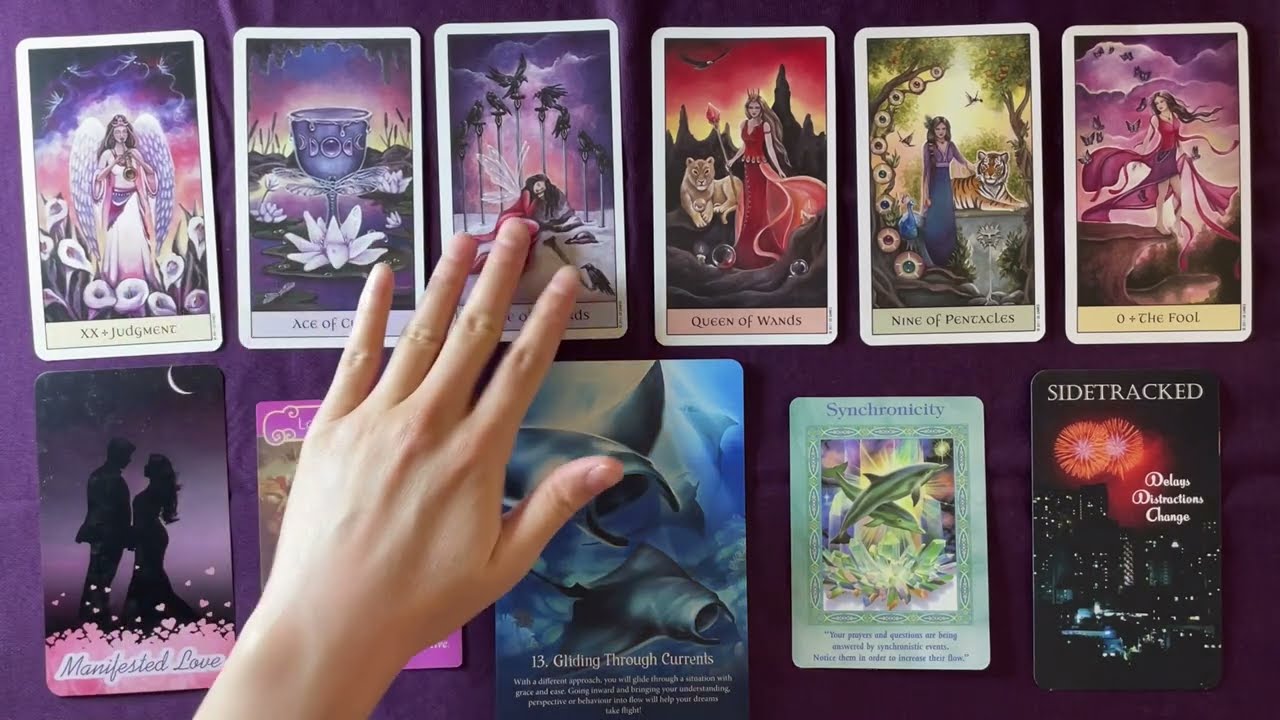In this horizontal photograph, a collection of 11 tarot cards is arranged on a purple cloth background. The cards are split into two rows, with six cards in the top row and five in the bottom. At the center, a white-skinned left hand is resting on the third card of the top row, partially obscuring its text and part of the second card as well. Each card prominently features a picture with text below it, primarily depicting women.

Detailing each card from left to right, the cards in the top row read: "XX plus Judgment," the text of the second card is partially hidden by the hand, the third card's text is obscured but lays below a woman lying down with trees in the background, "Queen of Pents," "Nine of Pentacles," and "Zero plus the Fool." The bottom row includes cards reading: "Manifested Love," the text of the eighth card is obscured by the hand, "Thirteen gliding through currents," "Synchronicity," and "Sidetracked."

Foreground elements like a glass utensil, dolphins, and a city highlight the varied and mystical imagery typical of tarot cards. The hand, extending from the left side of the image, adds a human touch to the scene, suggesting interaction with the cards.